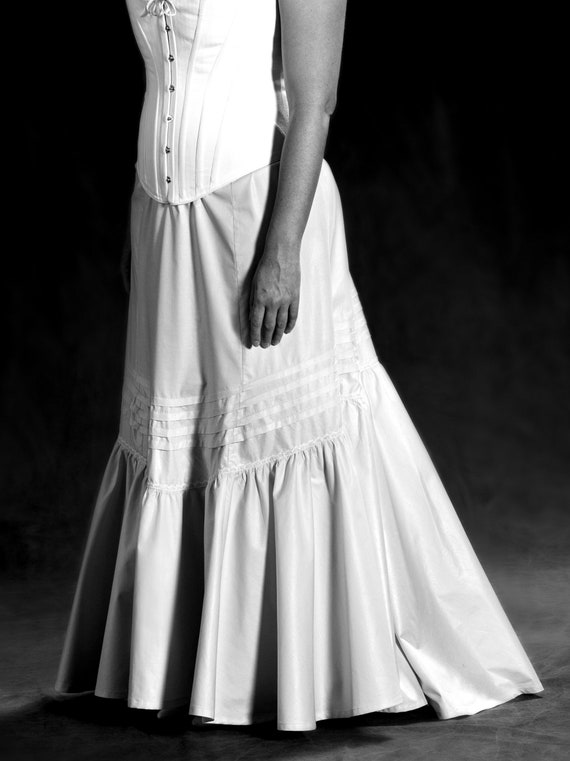The image is a black-and-white rectangular photograph set against a black wall and a gray floor. It features a woman dressed in period attire, captured from the mid-chest down. She wears a long, light-colored skirt that is very full and gathered at the bottom, with noticeable pleats and horizontal stripes about halfway down. The skirt appears to form a triangular point at the front before flowing into a more ruffled and gathered design. Her top is a form-fitting, corset-style white bodice with buttons running up the front and a small tie at the top. The bodice extends slightly over the upper part of the skirt. Only her left bare arm is visible, hanging down by her hip. Her feet and shoes are obscured by the fullness of the skirt.